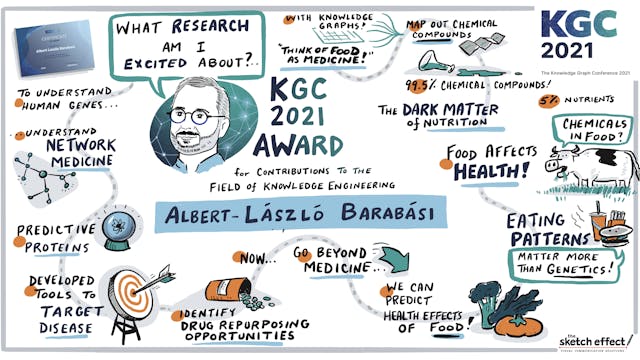The image presents a highly detailed, hand-drawn digital whiteboard, densely packed with colorful illustrations and text, set against a white background with a light gray border. Dominating the center and various parts of the image are themes related to knowledge engineering and nutrition.

In the upper right corner, in capital letters fading from blue to teal, it reads “KGC 2021,” which stands for Knowledge Graph Conference. Directly below this is a significant handwritten note, "KGC 2021 award for contributions to the field of knowledge engineering," indicating a special recognition.

In the center of the illustration, a light blue rectangle features the honoree's name, Albert-Laszlo Barabasi, spelled with accents over the "A" and "O" in Laszlo and over the second "A" in Barabasi. Directly above this rectangle is a circular illustration of a man with glasses, a beard, and short dark hair. A speech bubble from him asks, "What research am I excited about?" This figure emphasizes Albert-Laszlo Barabasi's pivotal role.

Surrounding these central elements are various interconnected illustrations and notes:
- In the upper left, an entry reads “Understand human genes” beside a blue card.
- Nearby, an arrow hits a bullseye with a note reading “Developed tools to target disease,” accompanied by a drawing of a target and an arrow.
- Further in the upper section, a note says, “With knowledge graphs, think of food as medicine, map out chemical compounds,” supplemented by illustrations like a beaker spilling chemicals and a notation “99.5% chemical compounds, 5% nutrients.”
- Another prominent element involves a cow's speech bubble asking, "Chemicals in food?" with surrounding notes stating “Food affects health” and “5% nutrients.” 
- The lower part of the image includes an illustration of a pill bottle underlined by the phrase “Identify drug repurposing opportunities” and a timeline noting “Go beyond medicine” with vegetable illustrations pointing towards predicting health effects of food.
- In the bottom right-hand corner, there's a mention of the Sketch Effect, potentially identifying the software used to create this illustration.

Overall, the image encapsulates the various aspects and achievements of knowledge engineering, prominently highlighting Albert-Laszlo Barabasi's contributions through a dynamic and visually engaging digital whiteboard.